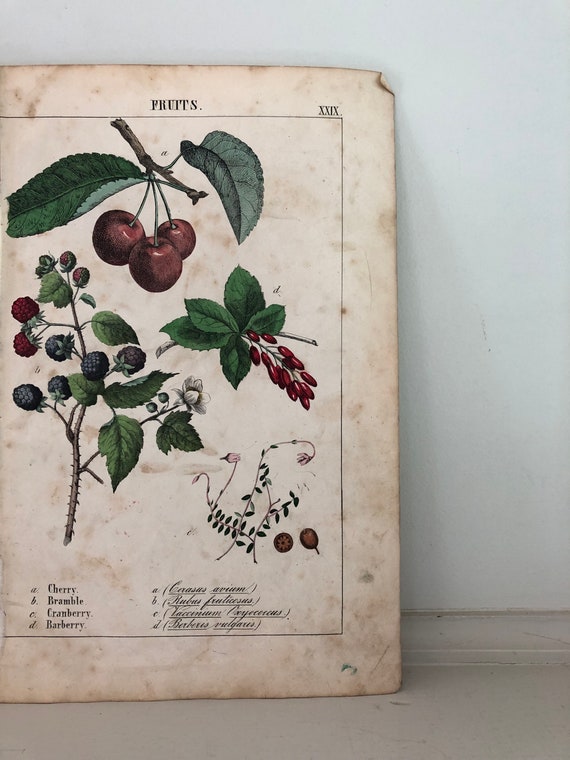The image shows a large, old, and dirty piece of paper that appears to have been taken from a book. The page, which is standing against a white, stained wall and resting on a concrete floor, is titled "Fruits" at the top. The upper-right corner of the page features the Roman numeral XXIX (29). The page is visually aged, with noticeable dirt and stains, and a small singe mark on the right-hand side. In the middle of the page, there are illustrations of various fruits, including cherries, blueberries, raspberries, and pomegranate seeds. Below these illustrations, the fruits are labeled alphabetically as A, B, C, and D with the names cherry, bramble, cranberry, and raspberry. The scientific or possibly Latin names of the fruits are listed but are not fully legible.